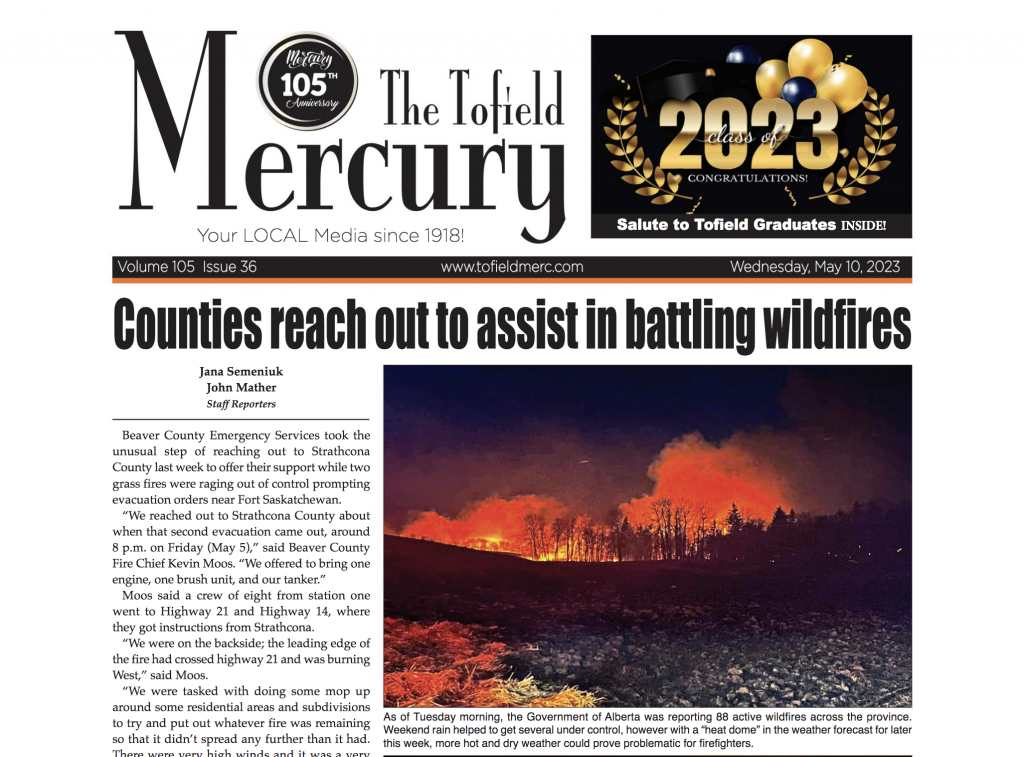This image showcases the front page of the Tofield Mercury's website, a long-standing local media outlet established in 1918. Dominating the right side of the page is a celebratory graphic for the Tofield High School Class of 2023. The design features a black square backdrop adorned with black and gold balloons and leafy decorations on either side. At the center, a circular emblem marks the 105th graduating class of Tofield High School, accompanied by a congratulatory message that reads "Salute to Tofield graduates inside."

This particular edition, dated Wednesday, May 10th, 2023, is volume 105, issue 36. It prominently headlines a report by staff reporters Jane Seamanluck and John Mayther about regional efforts to combat wildfires. The article describes how Beaver County Emergency Services extended aid to Strathcona County during two major grass fires last week. Complementing the article is a dramatic photograph of a grass fire, with dark smoke billowing into the sky, capturing the intensity of the scene. The website URL, www.tofield.com, is displayed, underscoring the paper's digital presence.